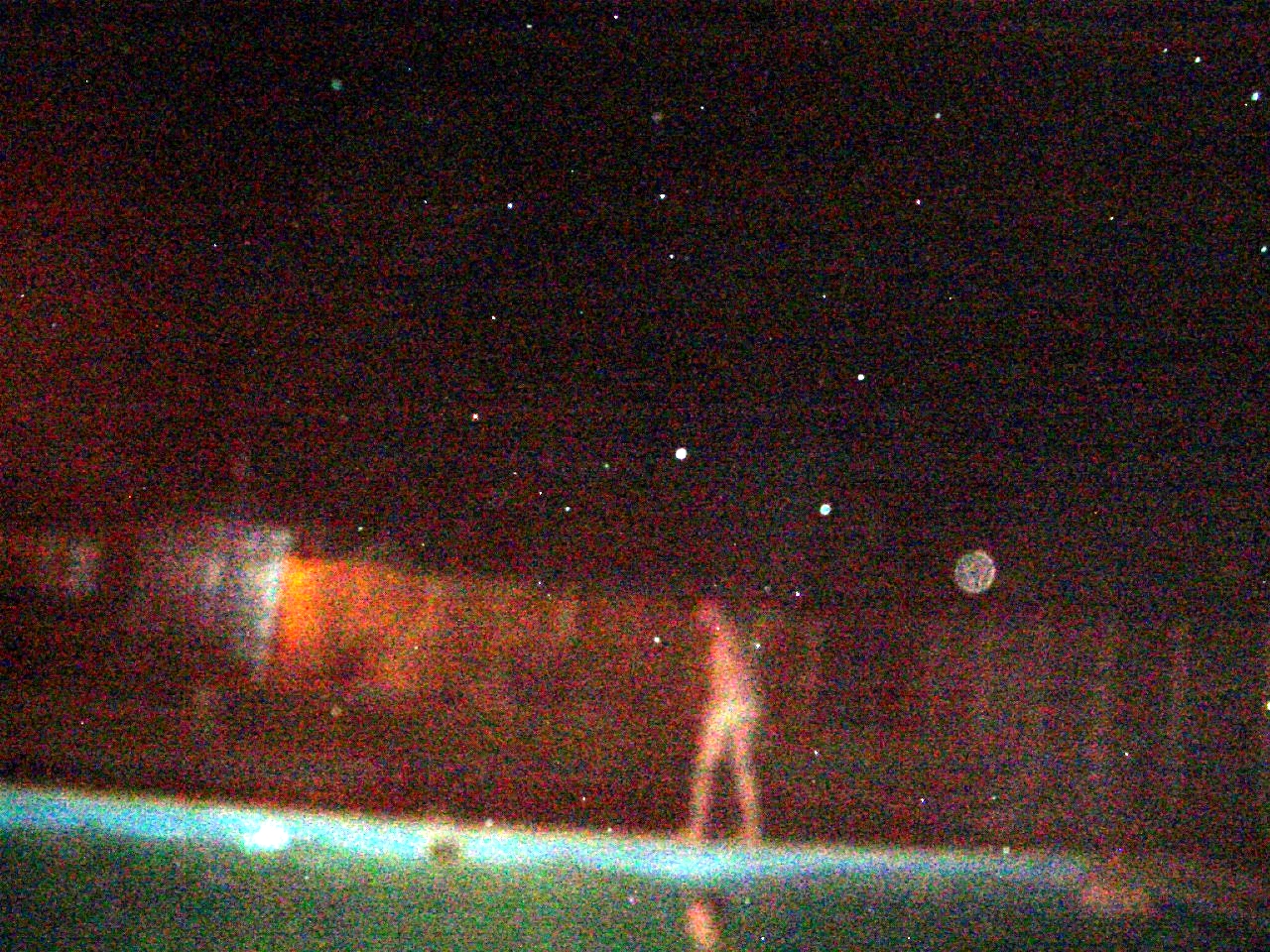This image is a photograph of an aged and damaged original photograph, characterized by noticeable blurriness, watermarks, and discoloration. The scene captures a rectangular pool with a blue liner, prominently featuring a pool filter return. In the pool, two Caucasian individuals are visible. Along the edge of the pool, a third Caucasian person is walking past, dressed only in white underwear. The setting is framed by a wooden privacy fence and a house in the background. The dark sky suggests that the photograph was taken at night.